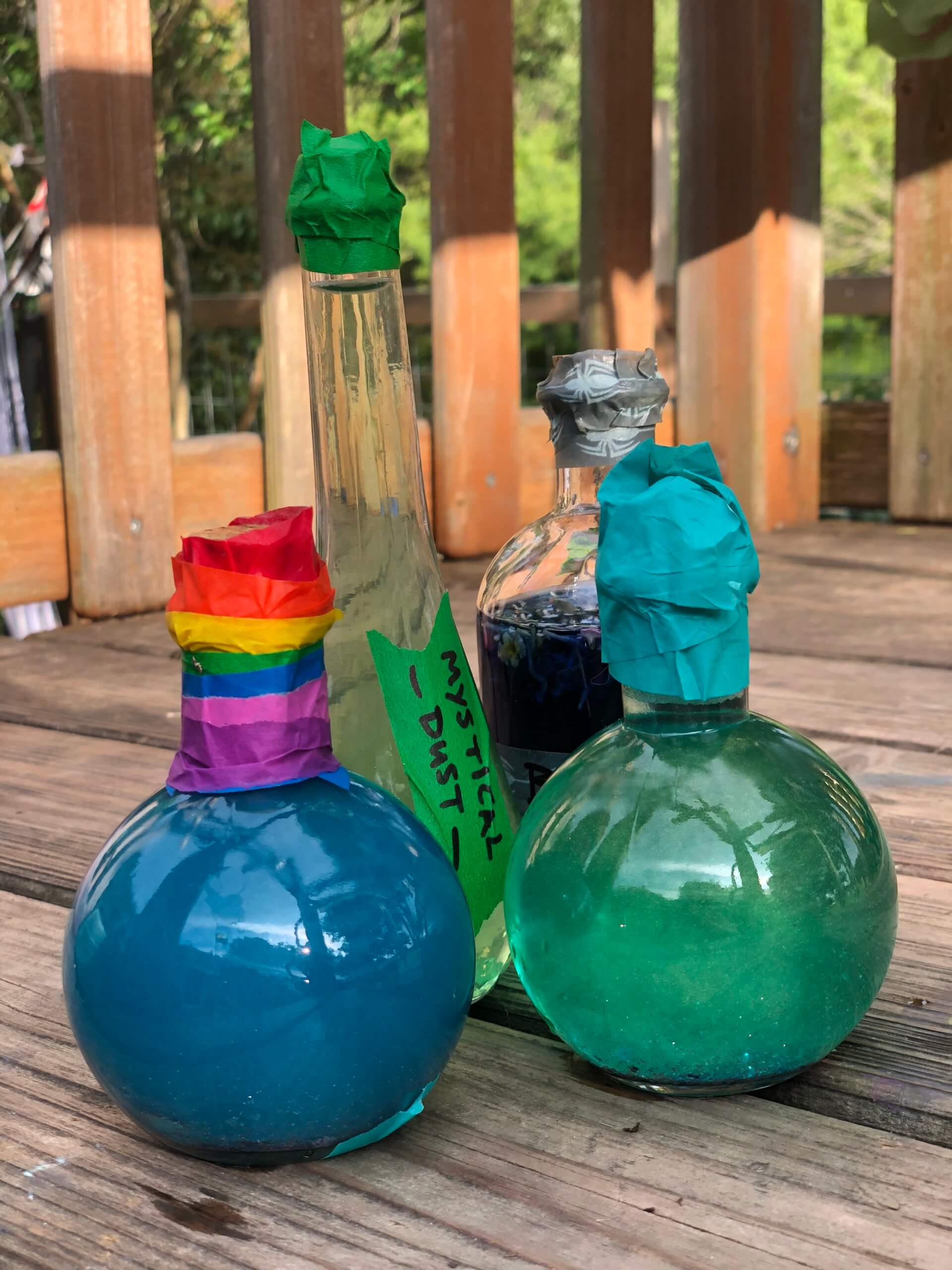The image depicts an outdoor scene on a deck, level with the floor, looking straight ahead towards a backdrop of green trees and a light brown railing. On the deck's wooden slats, there are four distinct bottles positioned in various arrangements. 

In the foreground, slightly to the left, is a round, bulbous bottle with a skinnier neck, sealed with paper that displays the colors of the LGBT pride flag. This bottle contains a dark blue liquid. To its right and slightly behind is a tall, slender bottle approximately twice as long, topped with green tape and labeled with a green sticker that reads "mystical dust." The label suggests an enigmatic content. Further back, there is a clear bottle with dark purple liquid inside, its top covered with silver tape. This bottle stands about two inches shorter than the slender one. 

To the far right of the image, another bulbous jar—similar in shape to the first one—has a teal blue tape around its neck, and inside it contains a greenish-blue liquid. Set behind all these bottles, there is a long, cylindrical vase-like container adorned with green tape around its neck, giving it a mystical appearance. The overall scene combines an air of mystery with vibrant color, creating a striking visual of oddly assorted ‘potions’ or concoctions against a tranquil outdoor backdrop.